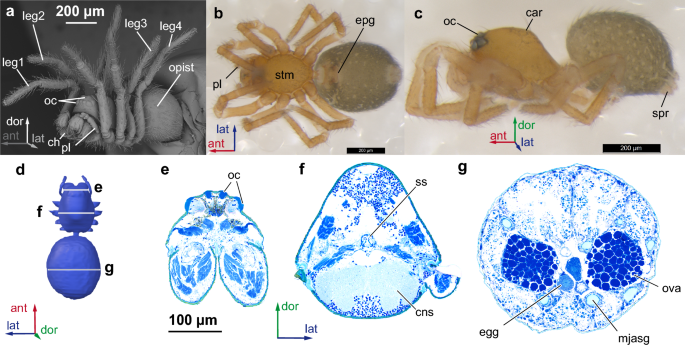The image is a detailed scientific diagram, similar to what you might find in a textbook or manual. It is a collage composed of several interconnected images of a spider. In the upper left-hand corner, there is a black and white photo or rendering of a spider, with its legs and other parts clearly labeled. This image is marked as A. To the right are two more labeled pictures of the spider; B shows a top view of the spider, featuring a tan front and a brownish circular stinger area, while C offers a side view, highlighting its crab-like legs and brown stinger area.

Beneath these images, from left to right, are computer-generated or x-ray-like scans of the spider, each labeled D through G. D is a 3D scan of the spider's body in a bluish hue. E is another scan, more medical in nature, resembling a blue x-ray. F continues with this blue outline x-ray style, and G delves into the internal structure, displaying the spider's egg or ova. All the images have specific labels and annotations, making the diagram highly informative and visually accessible.